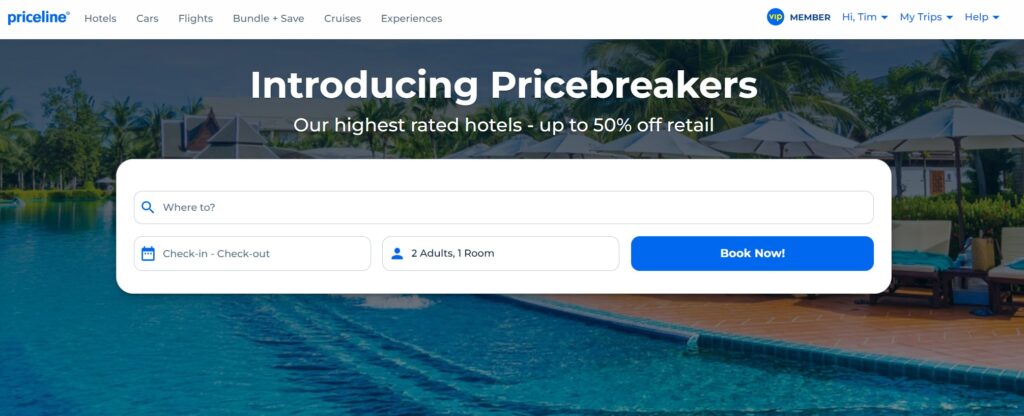This screenshot from the Priceline website features a clean layout with a white header bar at the very top. On the left corner, the Priceline logo is displayed in distinctive blue font. Adjacent to the logo, a grey font menu includes clickable options like Hotels, Cars, Flights, Bundle and Save, Cruises, and Experiences. On the upper right corner, user-focused options are available, such as Member, Hi Tim, My Trips, and Help, each presented as a dropdown menu.

Prominently displayed below the header is a vibrant photo of a luxurious pool scene. To the right side of the pool, there are cozy cabanas with umbrellas, framed by lush palm trees in the background. Overlaying this inviting image, in bold white text, is an enticing announcement: "Introducing Price Breakers. Our highest rated hotels – up to 50% off retail."

Directly beneath the photo, a sleek, white rectangular menu bar contains a search field. On the left of this field, there's a small blue magnifying glass icon, while the search field itself has placeholder text in black font that reads “Where To?” Below, there are selection buttons for Check-In and Check-Out dates, alongside a button indicating guest details: "Two Adults, One Room." On the far right, a prominent blue rectangle with white font stands out, urging visitors to “Book Now!”